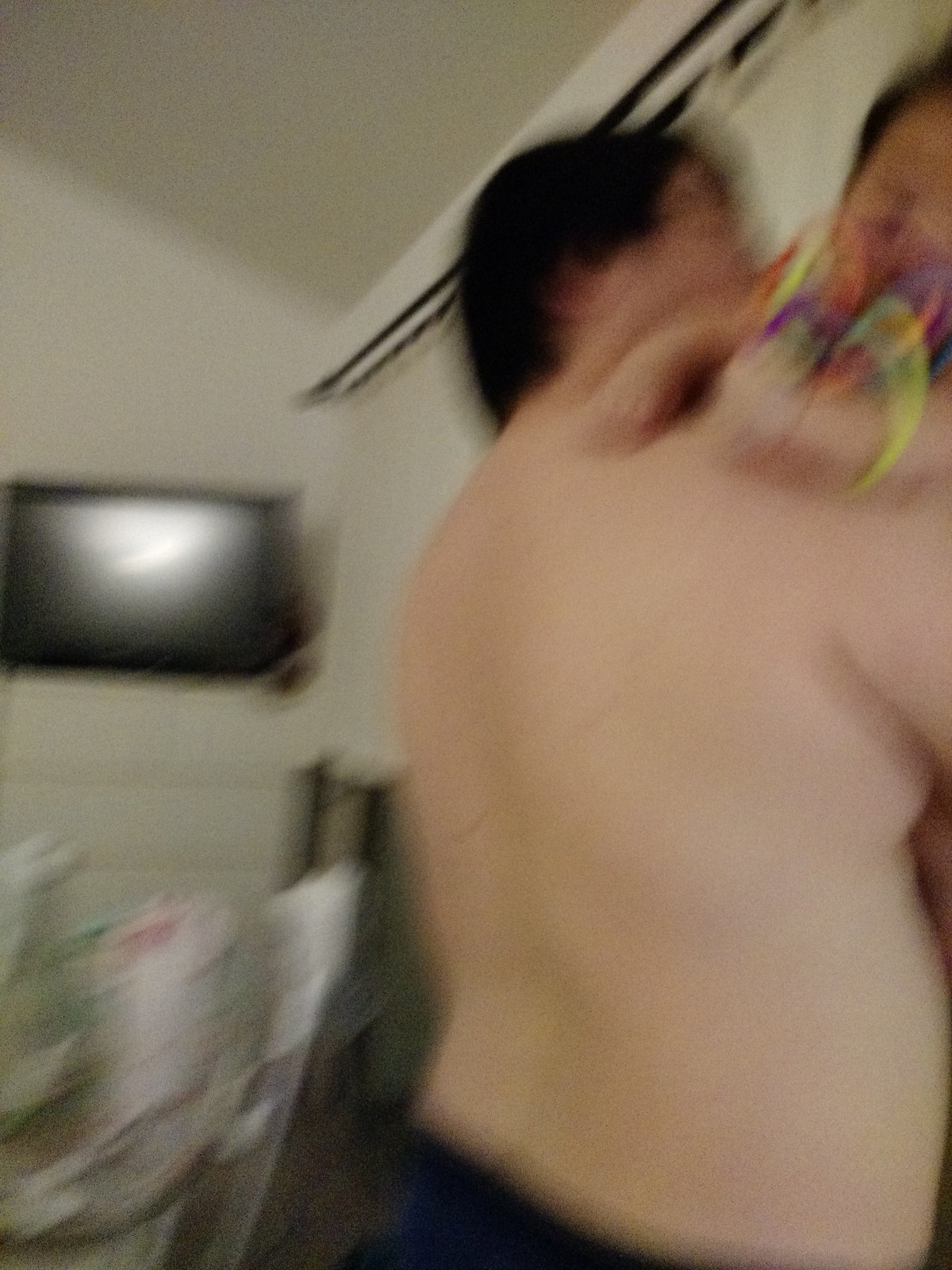In this very blurry image, a large, shirtless person with dark hair, possibly a man, is holding a small child, likely a toddler or baby, who has brown hair. The adult is located in the upper right corner of the picture and is wearing blue pants or shorts. The back of the adult is turned to the viewer, and they seem to be in a living room setting. The child, resting on the adult's shoulder, is holding a toy with distinct rings that are yellow, purple, and red. The background shows white walls, a curtain rod with white curtains, and a white dresser with three visible drawers. A small TV, approximately 32 inches, sits on top of the dresser. Additionally, a white stroller with green backing is positioned to the left of the adult, and a possible cot or playpen is visible at the bottom left of the picture. The ethnicities of the individuals are unclear due to the image's poor quality.